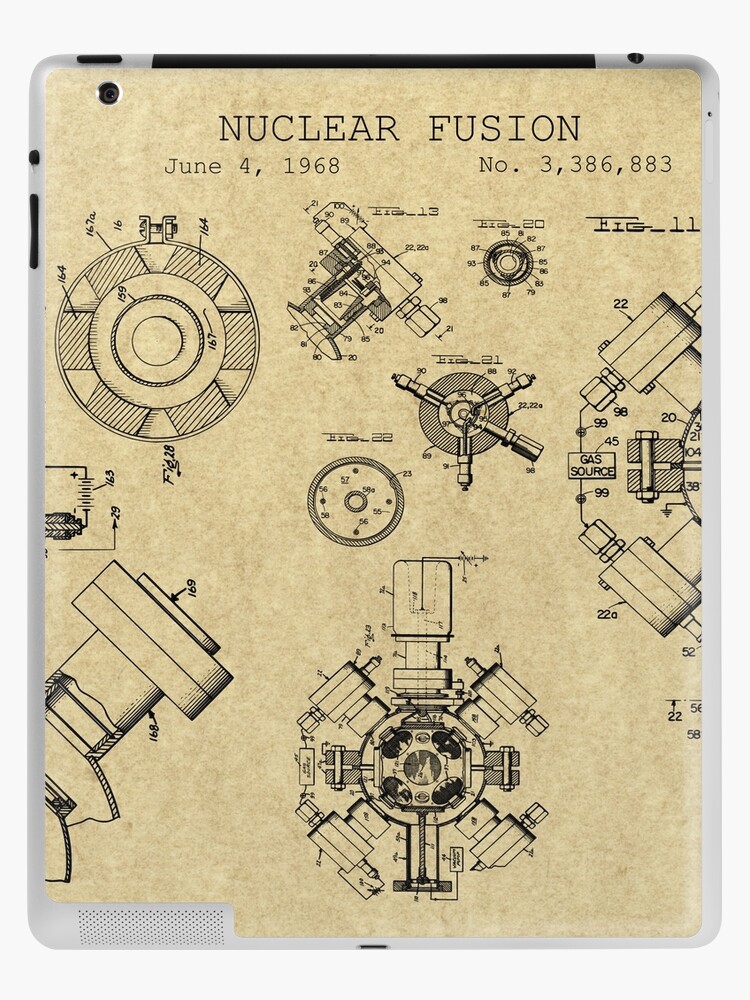This image displays what appears to be a vintage technical document or illustration, set against a tan background with black text. The heading at the top of the image reads "Nuclear Fusion," dated June 4th, 1968, and is labeled with the patent number 3,386,883. The document features a series of mechanical diagrams and illustrations, including a prominent white circle with dark, striped outer edges. Additional mechanical elements shown include what resembles a cordless or battery screwdriver, adjacent to an unreadable numerical dial and a black circle with a safe-like turning lock. Another diagram depicts a circle with a dark center, and there's an illustration that looks somewhat like a ship. The backing behind these illustrations seems to be a silver-colored frame, possibly suggesting it's part of a display or cover.